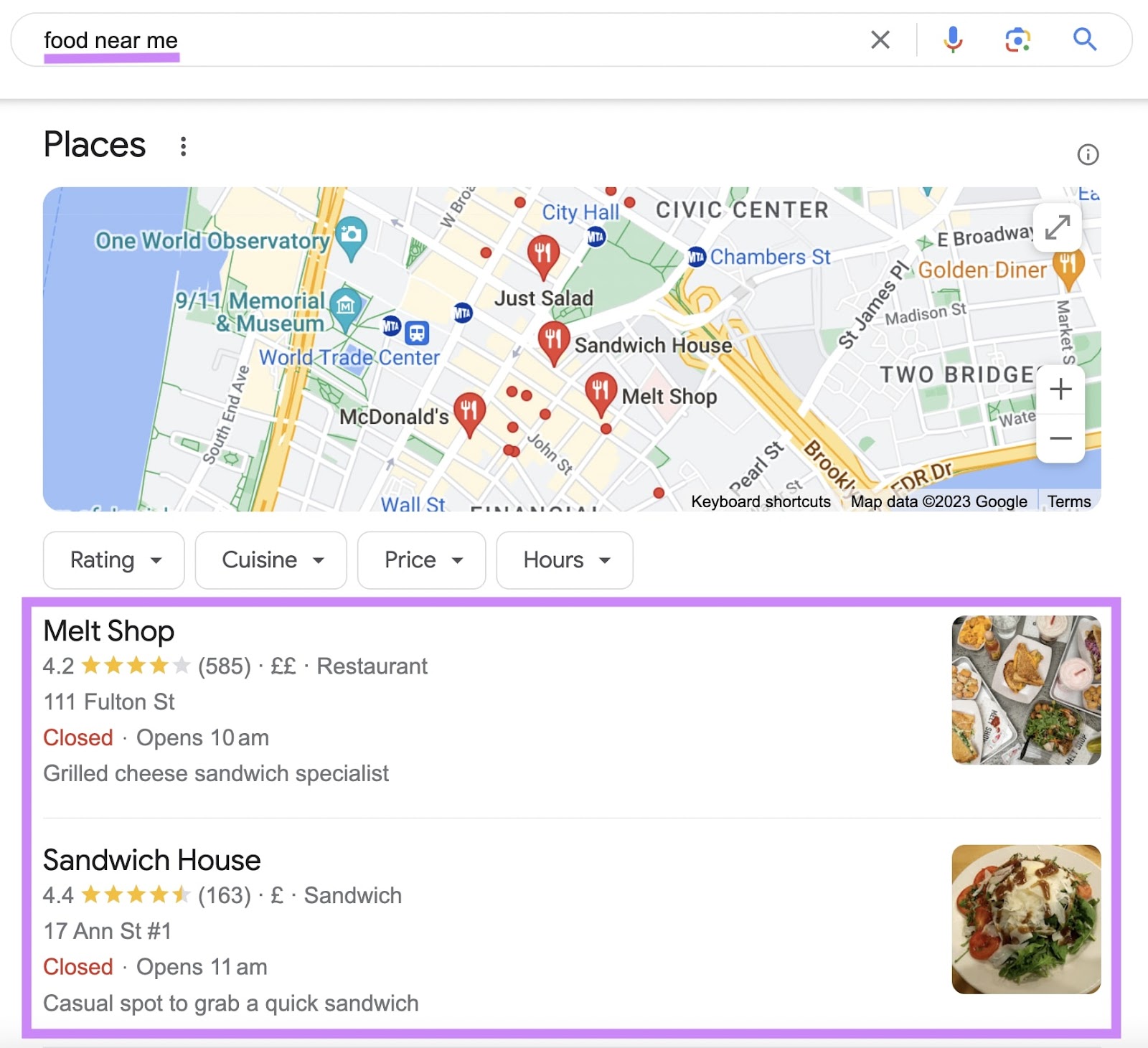The image is a screenshot showcasing search results for "food near me." At the top of the screenshot, there's a search bar flanked by icons for a microphone, camera (for image searches), and a magnifying glass (the search button). Below the search bar, the word "Places" indicates the category of the search. 

The map displayed in the middle segment has several red markers indicating food locations, though the specific geographic area is not identifiable. Beneath the map, there are multiple filter options shown as buttons and drop-down menus, labeled "Rating," "Cuisine," "Price," and "Hours."

Further down, the screenshot highlights the top two search results within a purple rectangle. The first result is "Melt Shop," which has a rating of 4.2 out of 5 stars based on 585 reviews. It is identified as a "Grilled Cheese Sandwich Specialist" and is marked with two pound signs (indicating moderate price). The location is specified as 111 Fulton Street, with the note that it is currently closed and will open at 10 a.m.

The second result is "Sandwich House," which boasts a rating of 4.4 out of 5 stars from 163 reviews. It has one pound sign (indicating a less expensive option) and is described as a "casual spot to grab a quick sandwich." The address provided is 17 Ann Street, number one. It is also noted to be closed at the moment, with plans to open at 11 a.m.